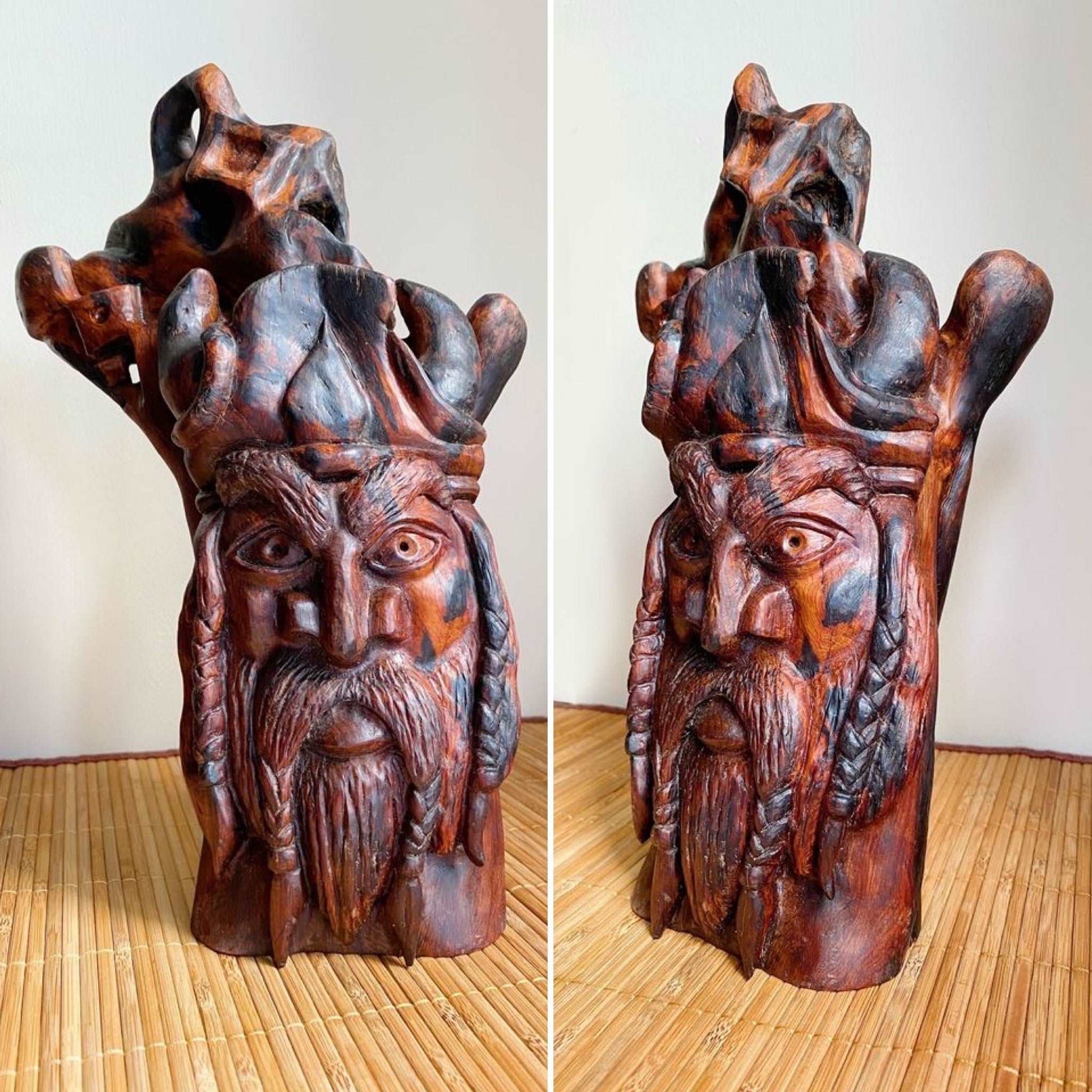The image features two side-by-side photographs showcasing a large wooden sculpture from different angles against a white wall, accentuating the sculpture’s dark features. The sculpture, carved from a single tree in a totem-pole style, presents a man-sized figure with a distinctly Viking-like face. Detailed with a heavy, long beard, the mustache is intricately braided at the ends, and the hair features elaborate braids along both sides of the face. His face has penetrating, large eyes, a prominent long nose with wide nostrils, and a slightly stern expression accented by small pupils.

The top part of the sculpture remains abstract, resembling a crown formed from the tree's original structure, stained dark brown with black and orange accents. Each photograph offers different perspectives: the left image shows a frontal view, highlighting the symmetry and details, while the right image reveals more of the figure's side profile, including the back of the head which has an object attached to it, suggesting a hat or bag. The entire sculpture rests on a bamboo floor, heightening the contrast between the dark wood and the bright background.